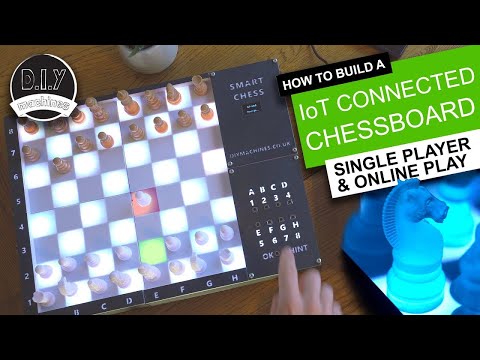The promotional screenshot serves as a detailed instructional guide on building an IoT-connected chessboard with options for single-player and online play. The background features a digital chessboard with a white and black checkered pattern, displaying a current game where white played E4 and black responded with B6. The board is surrounded by a colorful palette, including green, black, white, neon blue, dark blue, red, brown, and beige elements. Prominently, on the top right, the board is branded "Smart Chess." The top left corner showcases a logo labeled "DIY Machines." Additionally, there is a visible keypad for inputting chess moves using standard chess notation (letters A-H and numbers 1-8), towards which a hand is pointing. The predominant pieces on the board are white at the bottom and brown at the top, with a notable translucent blue horse piece among them. This comprehensive visual and textual presentation emphasizes the connectivity and modern functionality of the chessboard.